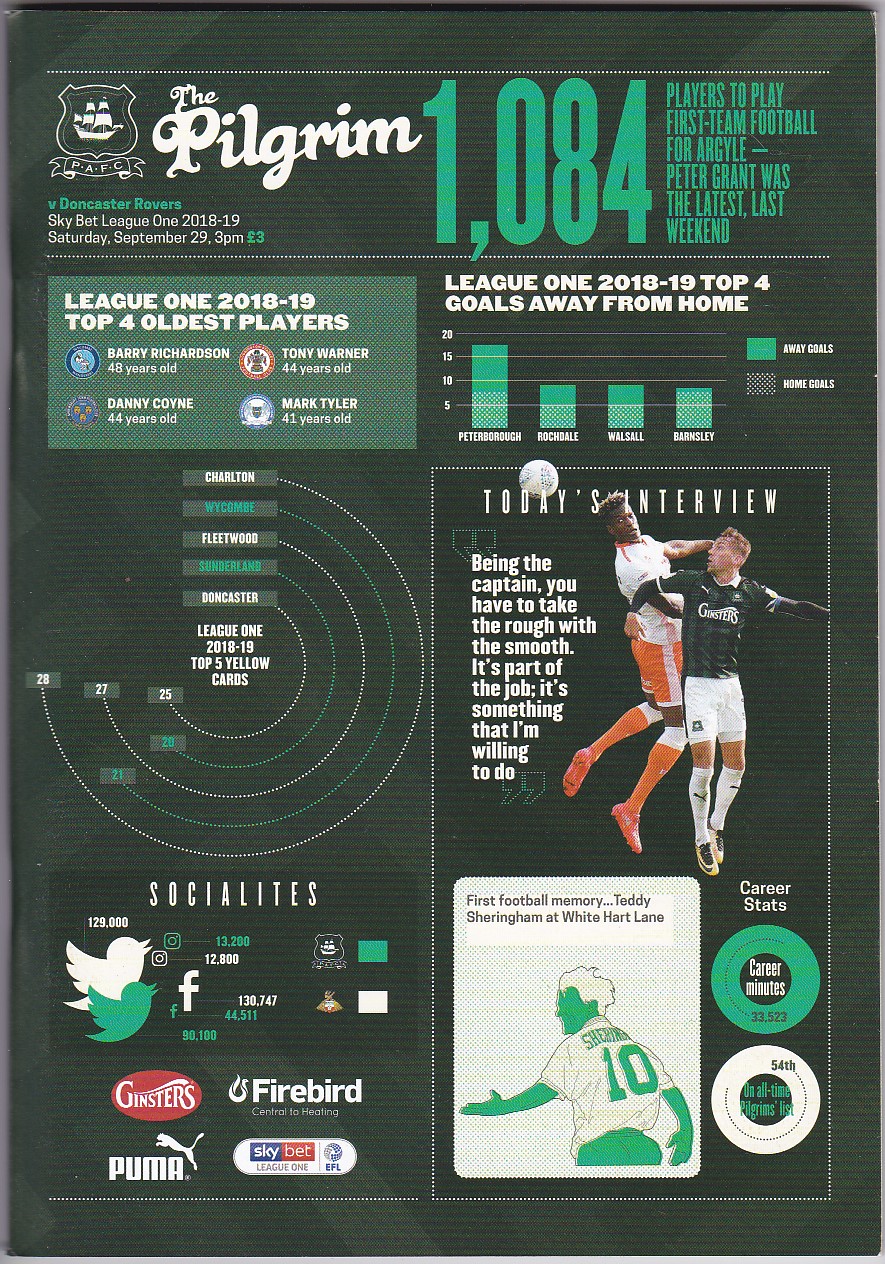This infographic presents an extensive array of soccer statistics and details for a league, themed predominantly in green, possibly mimicking a soccer field. Titled "The Pilgrim" in an old-style font at the top left, the header features a white clipper ship with a crest, and a banner reading "P.A.F.C." This section also includes "V. Doncaster Rovers" in green text, indicating a match, followed by "Sky Bet League One 2018-19" in white, the date "Saturday, September 29th, 3 p.m.," and a ticket price of "3-pound" in green. Directly to the right in large text is "1084," indicating the number of players who have played first-team football for Argyle, with Peter Grant being the latest player.

Beneath this header, the infographic is divided into several statistical sections. On the top left, a green square highlights the "League One 2018-19 Top 4 Oldest Players," listing each player with their respective team logos in color. Adjacent to this section, a bar graph titled "League One 2018-19 Top 4 Goals Away From Home" utilizes green bars for away goals and a screened effect for home goals.

Another section below features a unique circular infographic resembling orbital paths, showcasing the "League One 2018-19 Top 5 Yellow Cards," with player names and yellow card counts arranged along incomplete orbits. Further down, a segment labeled "Socialites" compares the social media followings of two clubs on Twitter, Instagram, and Facebook, with depicted logos and follower counts using green and white differentiation.

On the lower right, an interview section along with an action photograph of two soccer players contesting a header appears. Below this, a sketch of another player with the caption "First Football Memory: Teddy Sheringham at White Hart Lane" is detailed. Lastly, career statistics are visualized through circles showing "Career Minutes" and an "All-Time Pilgrims List," bordered with orbit-like paths displaying respective numerical data.

Overall, this visually engaging infographic combines a historic theme with detailed, color-coded soccer statistics to deliver a comprehensive overview of team and player performances in League One for 2018-19.